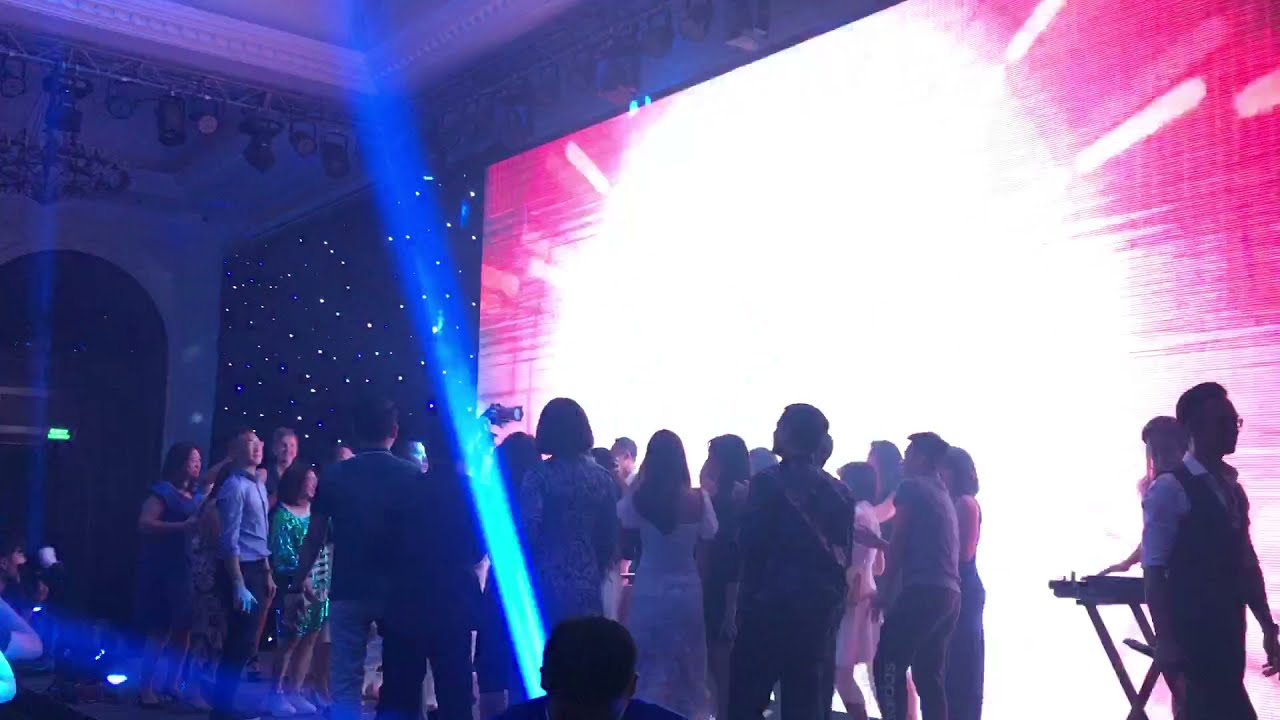The image captures a dark concert or demonstration with an otherworldly atmosphere. Dominating the scene is a large backdrop adorned with a neon pink design and a bright white center, from which white beams shoot out. The backdrop is illuminated by vibrant blue light running vertically, casting shadows of the people gathered in front. To the left of the neon pink display, there's a darker section speckled with what appear to be tiny, star-like flecks. The room is bathed in various neon hues, including pink, bright white, blue, purple, and teal, reminiscent of a galaxy. Spotlights along the ceiling cast additional light. Among the crowd, silhouettes of individuals can be distinguished, facing the backdrop and each other, with the majority having their backs to the camera. Notably, a man in the lower right corner appears to be wearing a suit without a jacket, next to other attendees dressed in blue and pink attire, adding to the vivid, surreal scene.